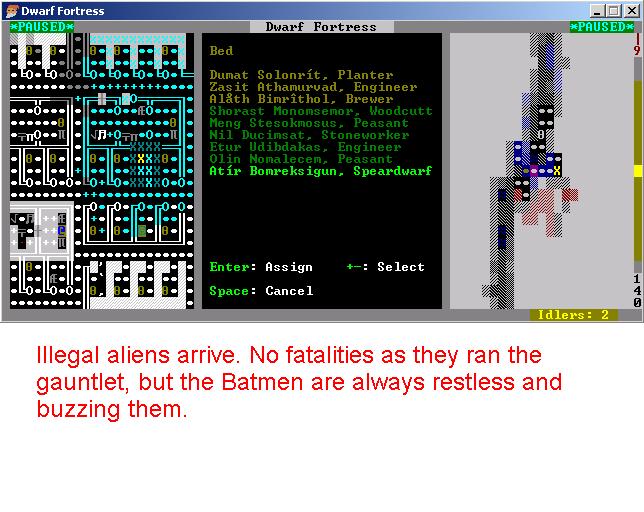The image, a computerized screenshot from an older version of the video game "Dwarf Fortress," showcases a divided interface. At the top, the title "Dwarf Fortress" is prominently displayed. The screen is split into three sections: on the left, a detailed blueprint-like layout of the fortress under construction; in the center, a list of dwarves along with their professions such as Planter, Engineer, Brewer, Woodcutter, Peasant, Stoneworker, and Spirit Dwarf; and on the right, what appears to be a map showing various elevations and possibly different rooms, indicated by pixelated graphics and assorted colors. At the bottom of the image, red text states: "Illegal aliens arrive. No fatalities as they ran the gauntlet, but the Batman are always restless and buzzing them."